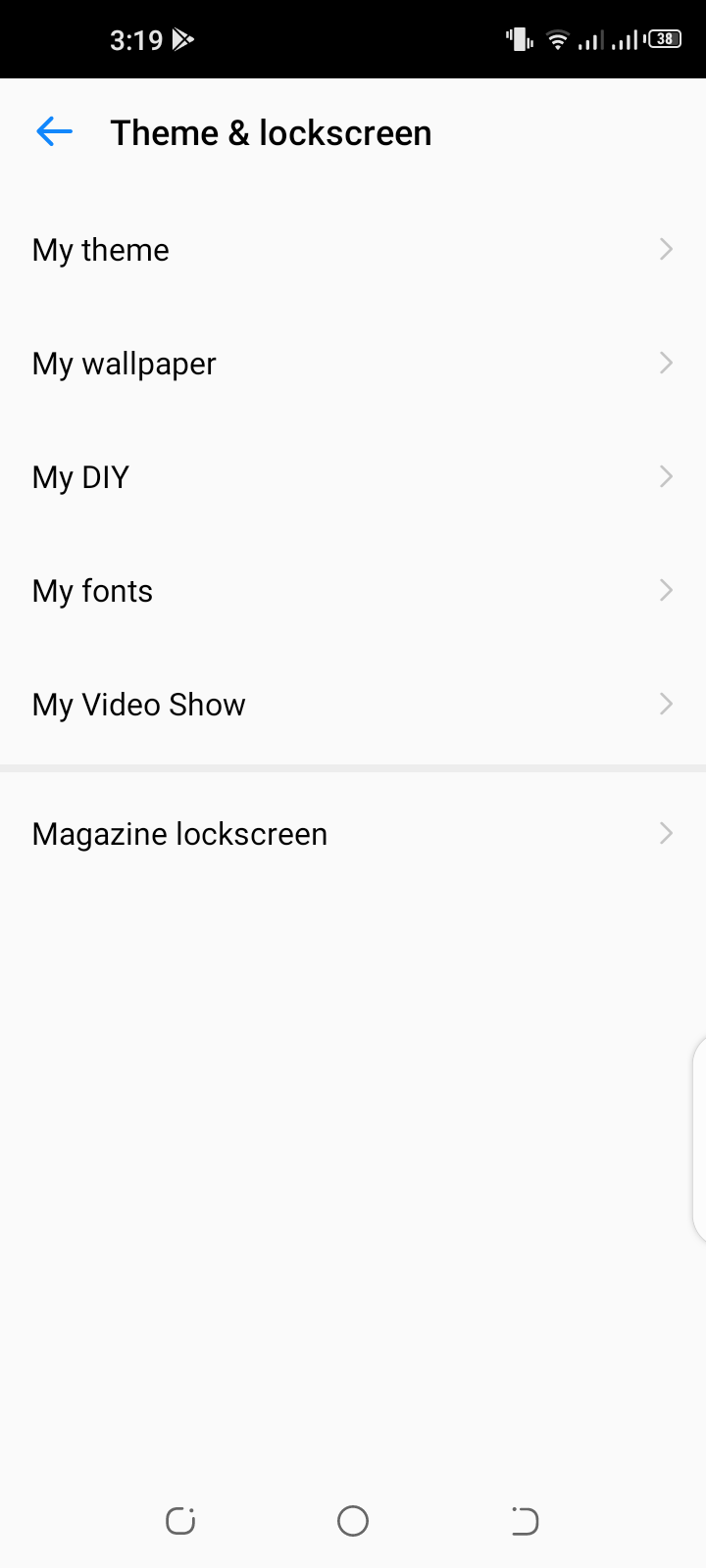Screenshot of a Mobile Device Displaying Theme and Lock Screen Settings:

At the top of the image, there is a black status bar displaying various pieces of information about the phone. In the upper left corner, the time is shown as 3:19 PM. To the right of the time, there are icons for the Play Store, and indicators for Wi-Fi (with 4 out of 5 bars) and 4G connectivity (with 3 out of 4 bars).

Beneath the status bar, there is a grey-themed settings screen with the heading "Theme and Lock Screen" displayed in black font. To the left of this heading, there is a small blue arrow, indicating a back or return function.

Below the heading, a list of clickable options is presented, each with a small grey arrow on the right side to suggest further navigation. The options listed are as follows:
1. My Theme
2. My Wallpaper
3. My DIY
4. My Fonts
5. My Video Show

Between the list of options and the next section, there is a light grey separator line. Below this separator is another clickable option labeled "Magazine Lock Screen."

At the bottom of the screenshot, typical mobile navigation icons are visible:
- A back arrow on the left
- A home screen icon in the center
- A minimize or multitask button on the right

The overall layout and design elements, such as the status bar, navigation icons, and clickable settings options, indicate this is a screenshot taken from a mobile device.